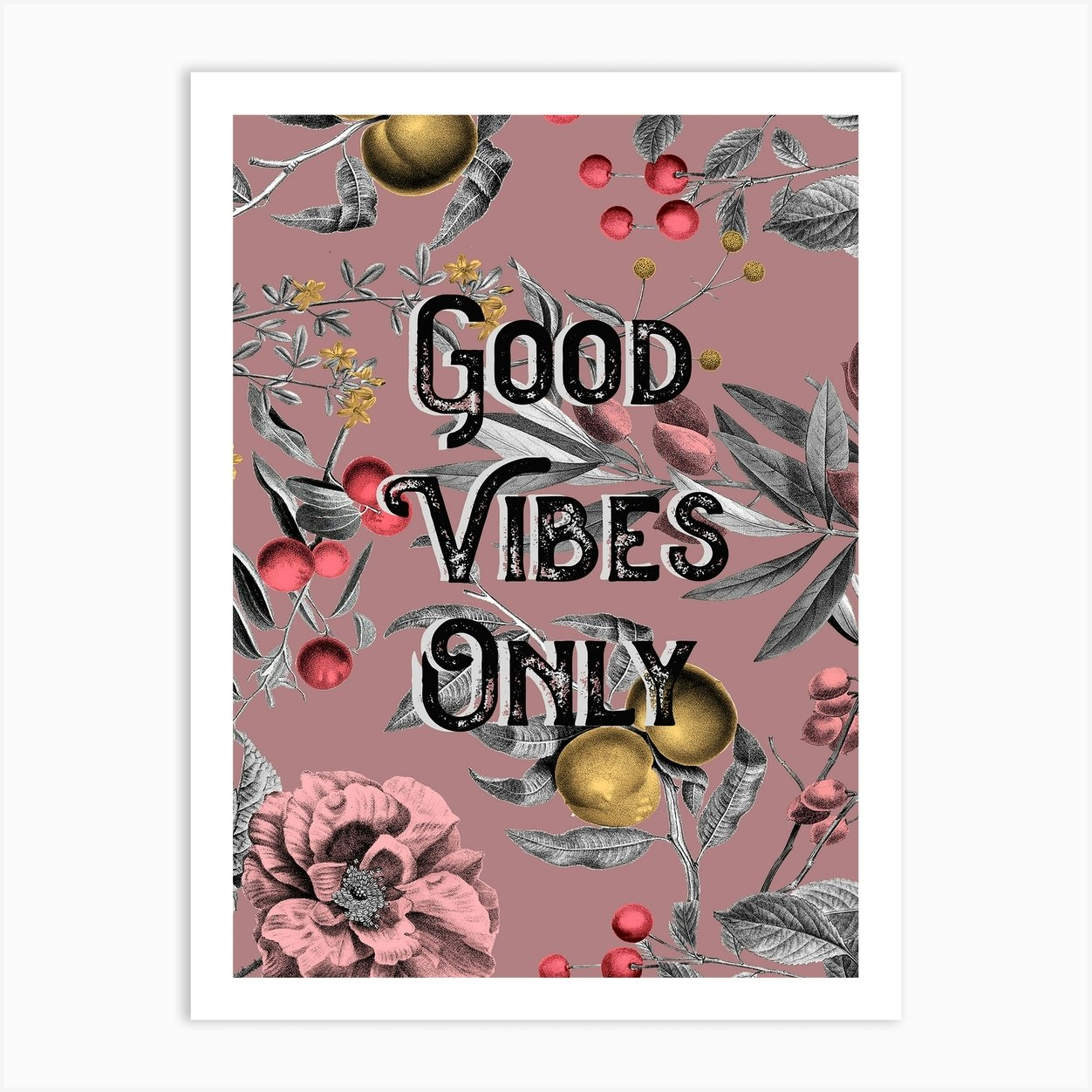This square piece of motivational artwork features the phrase "Good Vibes Only" prominently displayed in embossed gray and speckled gray lettering, with the 'G' and 'V' capitalized, on a dusty pink background. The image is framed in white and photographed against a white wall. The background of the artwork includes delicate illustrations of gray leaves, twigs, and vibrant red berries, creating a serene, nature-inspired scene. In the bottom left corner, a large pink flower with a gray center adds a soft, elegant touch, while on the bottom right, a stalk with gray leaves bears two tan orbs, likely representing fruit. The hand-drawn or potentially digitally designed elements give the artwork an artistic and hand-painted feel, enhancing its charming and motivational aesthetic.